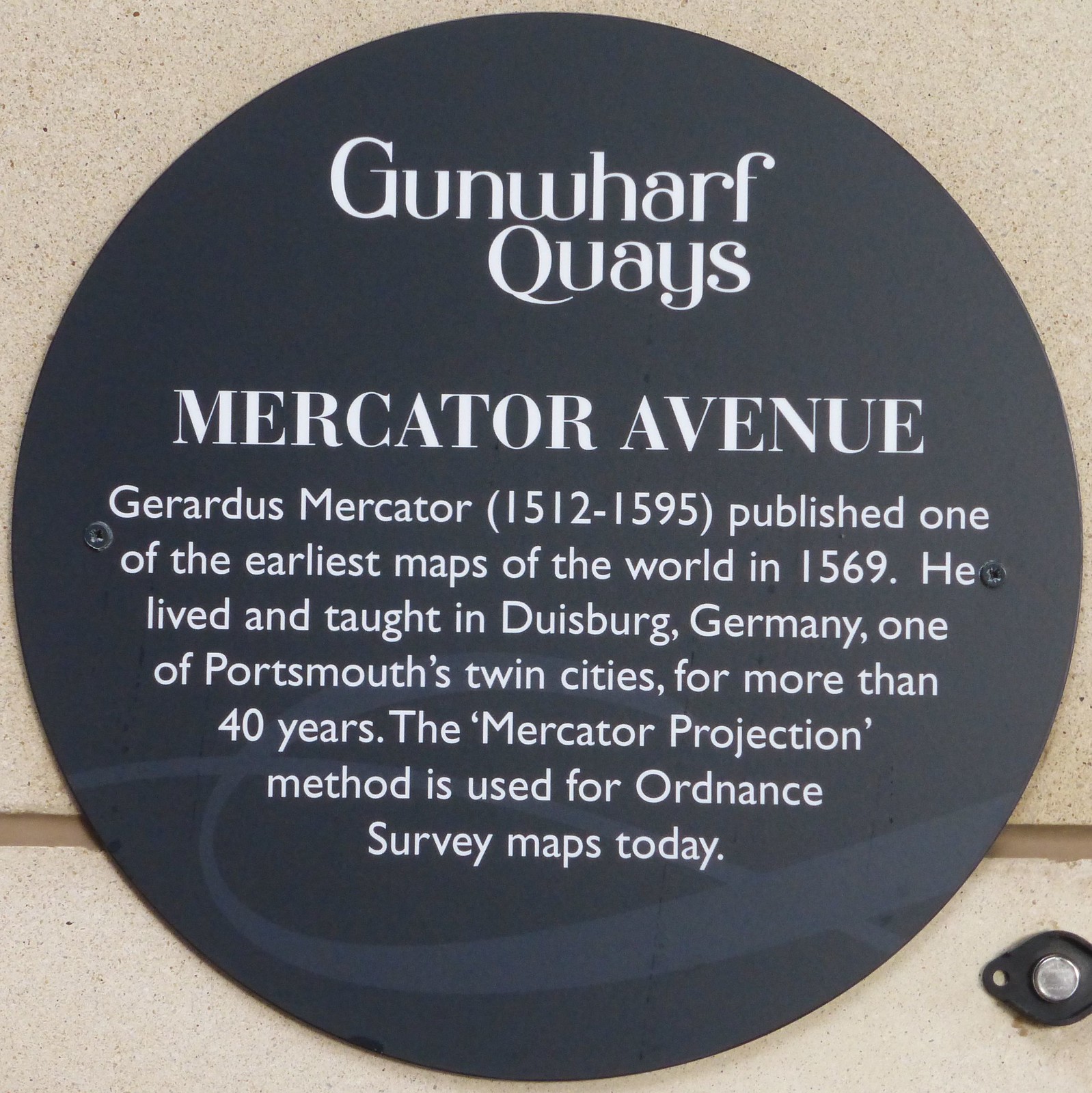The image features a square plaque mounted on a beige wall with thick beige tiles and brown cement separating them. The plaque itself is navy blue with a circular shape and two screws on either side. At the top in white font, it reads "Gunwharf Quays." Below that, in all capital letters, it says "Mercator Avenue." The main text following this heading states, "Gerardus Mercator, 1512-1595, published one of the earliest maps of the world in 1569. He lived and taught in Duisburg, Germany, one of Portsmouth's twin cities for more than 40 years. The Mercator projection method is used for ordinance survey maps today." The plaque also features a slightly lighter blue pattern at the bottom.